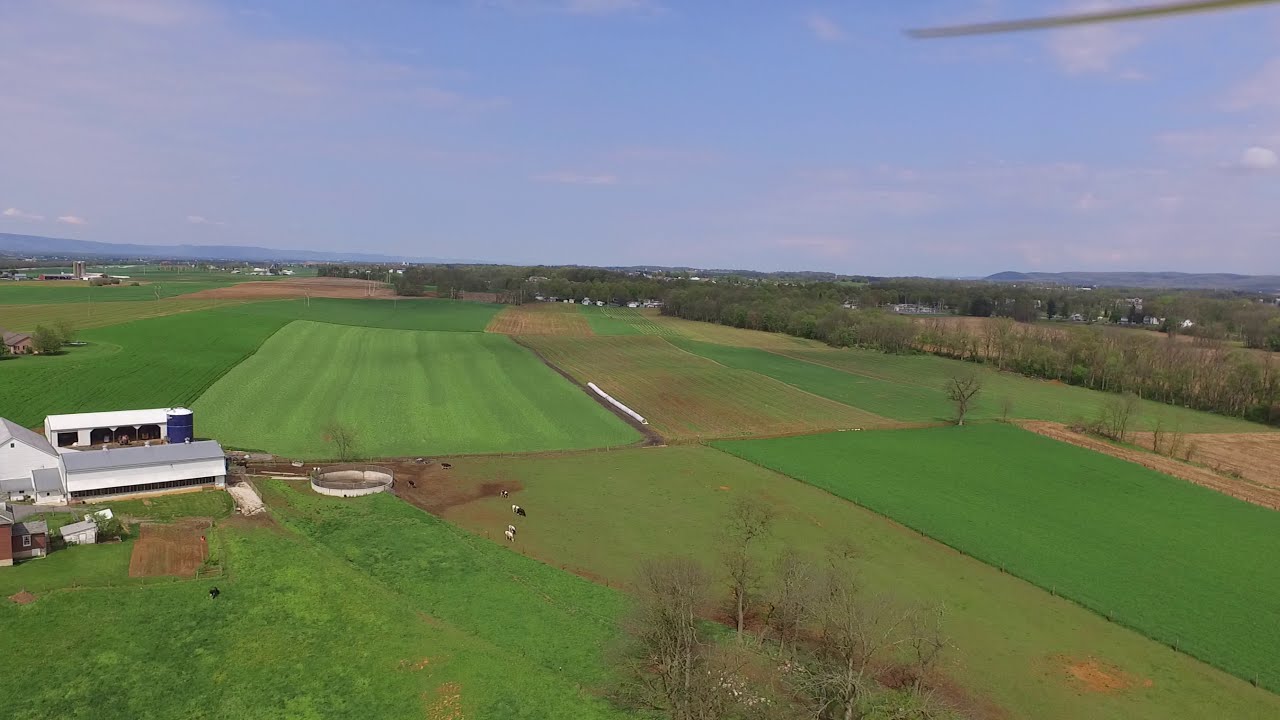This overhead aerial photograph, likely captured from a low-flying plane or drone, showcases a vast expanse of American Midwest farmland. The landscape is divided into multiple rectangular and square plots of land, predominantly green with some patches of light green and brown, which may indicate recently planted crops or seasonal variations. Centrally located in this agricultural expanse, these neatly sectioned fields hint at a well-organized farming system.

To the left side of the image, there are several structures forming a small cluster. These buildings include a prominent white barn with a triangular roof, accompanied by a longer barn to its right, both serving as likely storage or equipment areas. Additionally, a large blue cylindrical silo, possibly for grain storage, stands nearby, enhancing the agricultural ambiance of the scene. Scattered trees provide a natural boundary around this farming area.

In the background, the scenery transitions into a lush, wooded area with tall, bushy trees. Farther in the distance, one can discern large black mountains juxtaposed against a clear blue sky, adding a majestic backdrop to the rural setting. Extending towards the right side of the image, additional warehouse-like buildings are visible along with rolling hills or smaller mountains. The intricate details, including a potential glimpse of a plane propeller at the upper right, underscore the expansive and meticulous nature of this beautifully captured farmland.